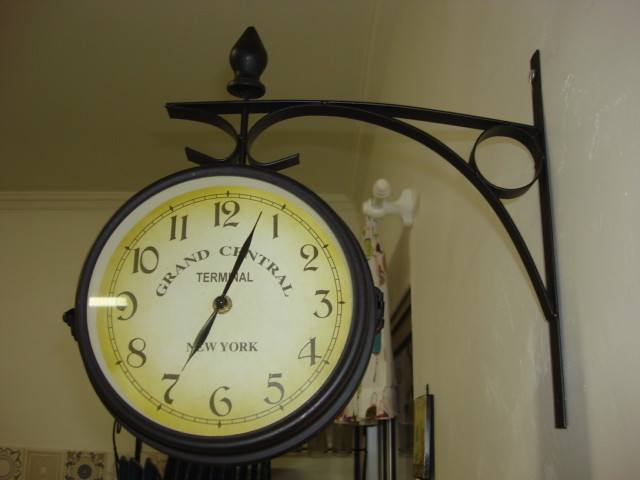This rectangular landscape image, approximately 20% wider than it is tall, captures a clock situated inside a terminal. The clock is prominently displayed, mounted on an ornate black iron bracket that juts out from a wall on the right side of the frame. The wall, along with the ceiling and back wall, are all painted in an off-white, yellowish cream color, though the overall lighting in the scene is relatively dim.

The iron bracket supporting the clock is intricate, featuring a vertical iron bar that extends much of the height of the image. This vertical bar is connected to a horizontal bar by a curved brace, forming a design that includes an iron circle nested within a triangular shape created by the three bars. Other ornate details contribute to the elaborate metalwork, from which the round clock is suspended.

The clock itself has a black iron frame and is positioned slightly left of center in the image, angled somewhat to the left rather than facing directly forward. Its face is a light yellow, shielded by glass that reflects sunlight, noticeable particularly around the nine o'clock position. The clock displays standard numbers from one to twelve. The time shown is approximately four minutes past seven, indicated by thin, pointed hour and minute hands.

Around the upper portion of the clock face, the words "GRAND CENTRAL" are written in all caps, following the curve of the clock. Directly below that, the term "TERMINAL" is written. Beneath the center, partially obscured by the hour hand, the text "NEW YORK" is visible, completing the description on the timeless face.